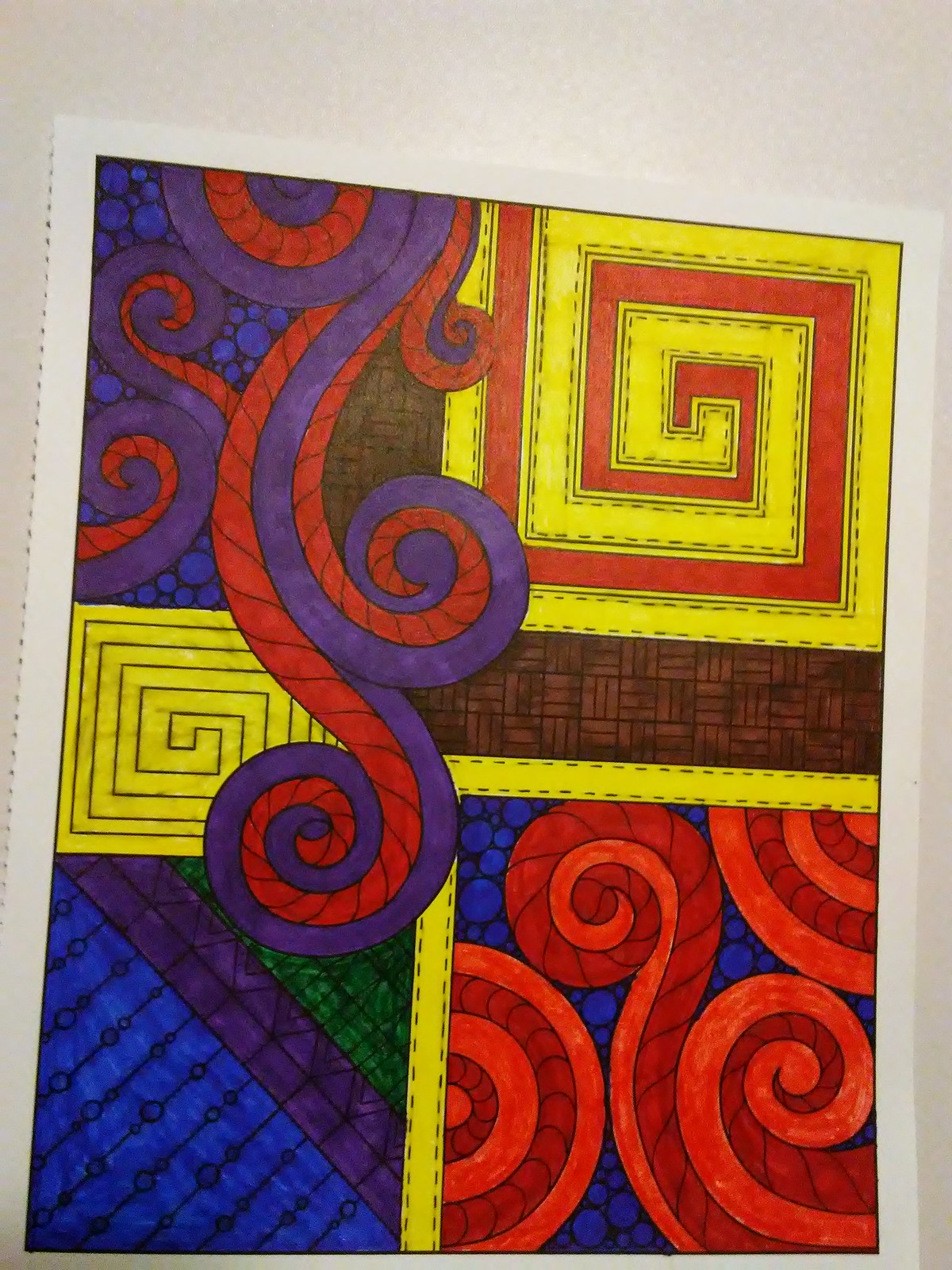This image depicts a colorful, tapestry-style drawing done in marker on a sheet of white paper, which appears to have been taken from a coloring book, as indicated by the perforated left edge. The drawing consists of several distinct sections, each with its own unique design and vibrant color scheme. The upper right-hand corner features interlocking geometric square spirals in bright orange and yellow, creating a mesmerizing inward pattern. Adjacent to this on the upper left are large, flowery swirls in purple and red, adding a sense of whimsy and movement. The lower left section showcases a mix of blue with black lines, green, and purple, woven with pink or purple stripes, somewhat reminiscent of trim patterns found on buildings. Finally, the bottom right corner is dominated by red and orange swirls surrounded by blue dots. This intricate and colorful creation has been captured in a top-down photo, suggesting it might be displayed on a flat surface like a counter or even tacked onto a refrigerator.